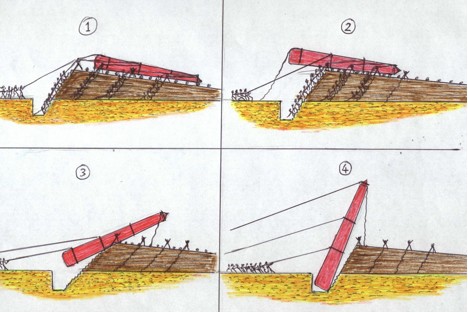The rendered image illustrates a detailed step-by-step process for erecting a large red pillar using a pulley system, shown through four distinct panels arranged in a two-by-two grid. Each of the panels is labeled with numbers 1 through 4, encircled, and separated by plus signs. The boat-like base they are working on has a yellowish-brown color, with the main deck being brown. 

In panel 1, stick-figure people are pulling on ropes with the red pillar laid horizontally above the brown deck area. Moving to panel 2, the pillar is being gradually pulled towards them, hanging slightly off the ledge. In panel 3, the pillar is tilted downward into an indentation in the middle of the deck. Finally, in panel 4, the pillar stands almost upright within the indentation, as the people hold the bottom ropes to secure it in place.

The visual sequence effectively demonstrates the meticulous process by which the stick-figure individuals maneuver the heavy pillar using ropes and a pulley system on what seems to be a boat, giving a clear depiction of the coordinated effort required for erecting the structure.